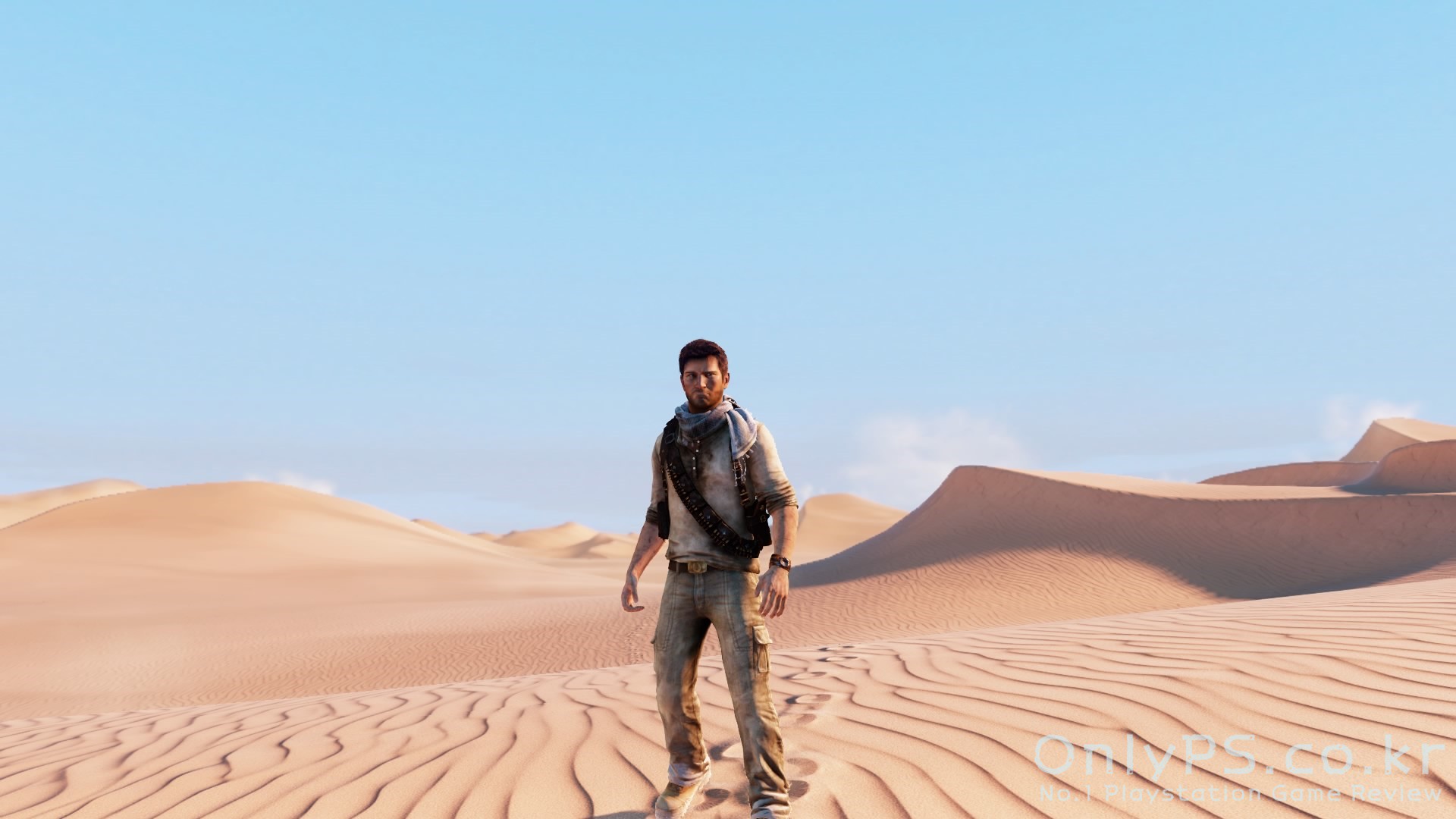The rectangular screenshot from a video game displays a rugged 3D-rendered man standing prominently in the center, facing forward. Dressed in khaki-colored cargo pants with side pockets and flaps, tan boots, and a white long-sleeve shirt with sleeves rolled up to his elbows, the figure exudes a weathered, sandy appearance, especially along the edges of his clothing. He has short brown hair and features accessories such as a wristwatch on his left wrist and a white scarf around his neck. Adding to his rugged look is a strap over his shoulder and torso, indicating the presence of a backpack partially visible behind his arm. The background portrays expansive tan-colored sand dunes beneath a blue sky with a single white cloud. The overall desert setting enhances the character’s gritty, survivalist aura. Additionally, white text reading "only ps.co.kr" is situated in the lower left corner of the image, though some of it is too faint to be legible.